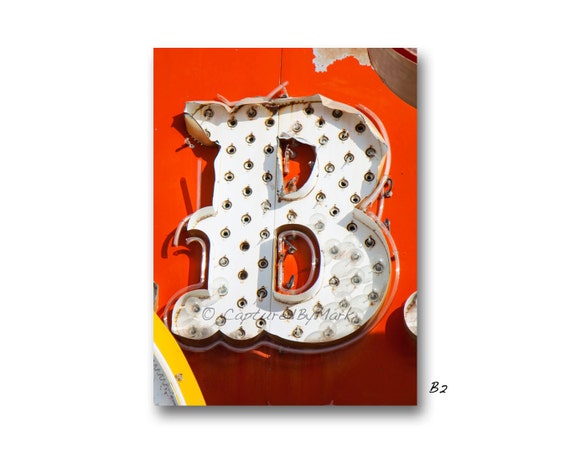The image depicts an ornate letter 'B' commonly found in vintage carnival or circus signage, featuring numerous sockets designed for light bulbs, giving it a nostalgic, old-timey appearance. The 'B' is white and prominently set against a red background, which varies in shade from brighter at the top to darker at the bottom, possibly due to shadowing. The background is notably worn and peeling, revealing patches of white and adding to the antiquated feel of the scene. A watermark indicates the photo is copyrighted by Mark. Additional details in the image include an oval-shaped yellow object in the bottom left, a brownish-red, splotched area in the top right corner, and a notation marked "B2" at the bottom right. The overall setting gives the impression of an abandoned carnival or circus sign that has weathered the passage of time.